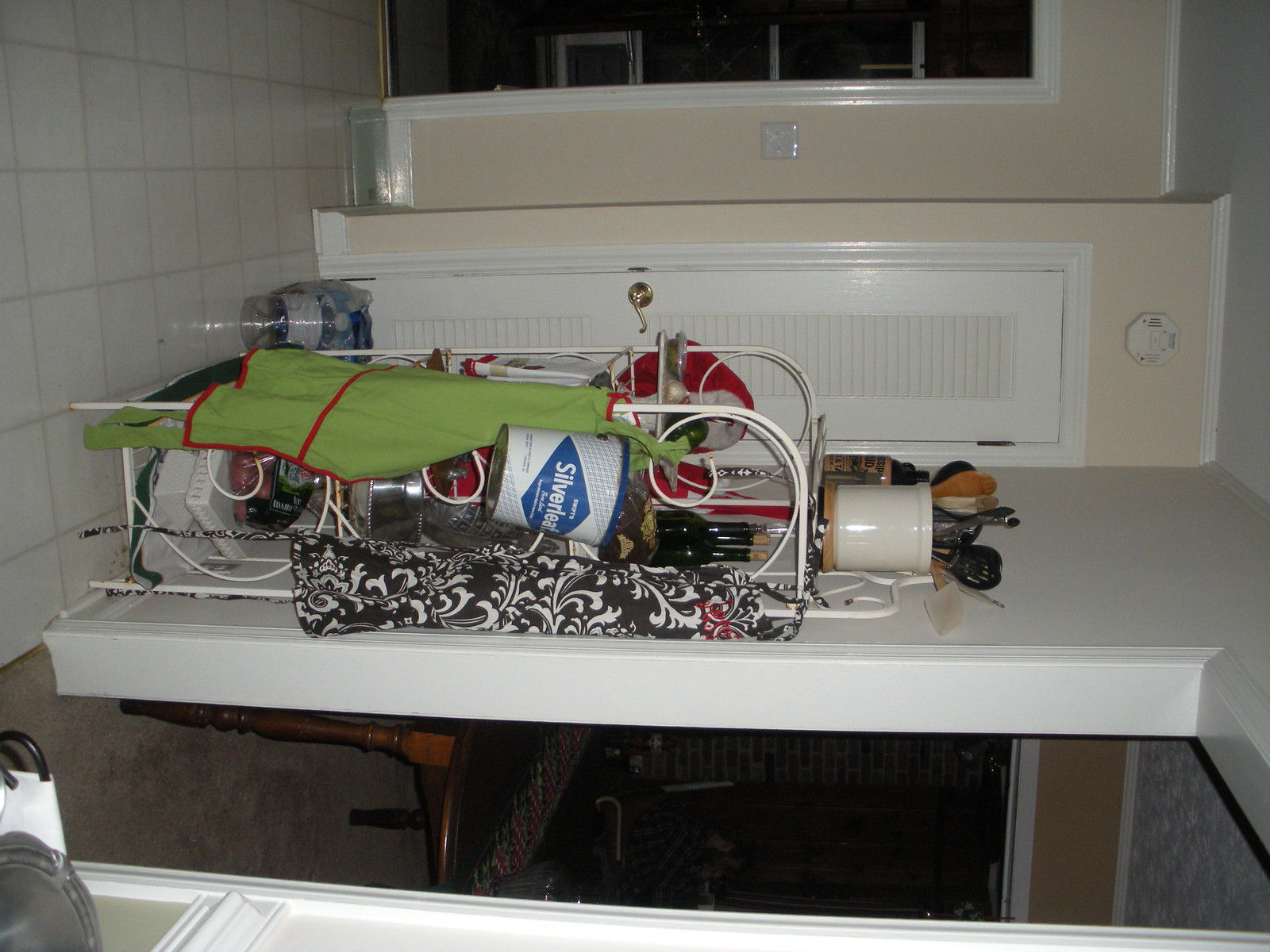On a white tabletop, a variety of objects are scattered, creating a scene of organized chaos. Resting on its side, a metal rack with intricate scrollwork is positioned to give the impression that the floor is actually the wall due to a 90-degree rotation of the image. At the top of this rack, there’s a ceramic utensil holder brimming with kitchen tools. Nestled on one of the shelves, a bottle of silver polish is clearly visible. Behind the rack, a pantry door stands slightly ajar, offering a glimpse of another room beyond it. Closer to the viewer, a doorway frame interrupts the pristine white backdrop, emphasizing the cohesive color scheme of white walls, trims, and floored surfaces. Adding a splash of color and texture, two pieces of fabric—a vivid lime green and a white one with a paisley pattern—are draped casually on the table, enhancing the visual interest of the scene.